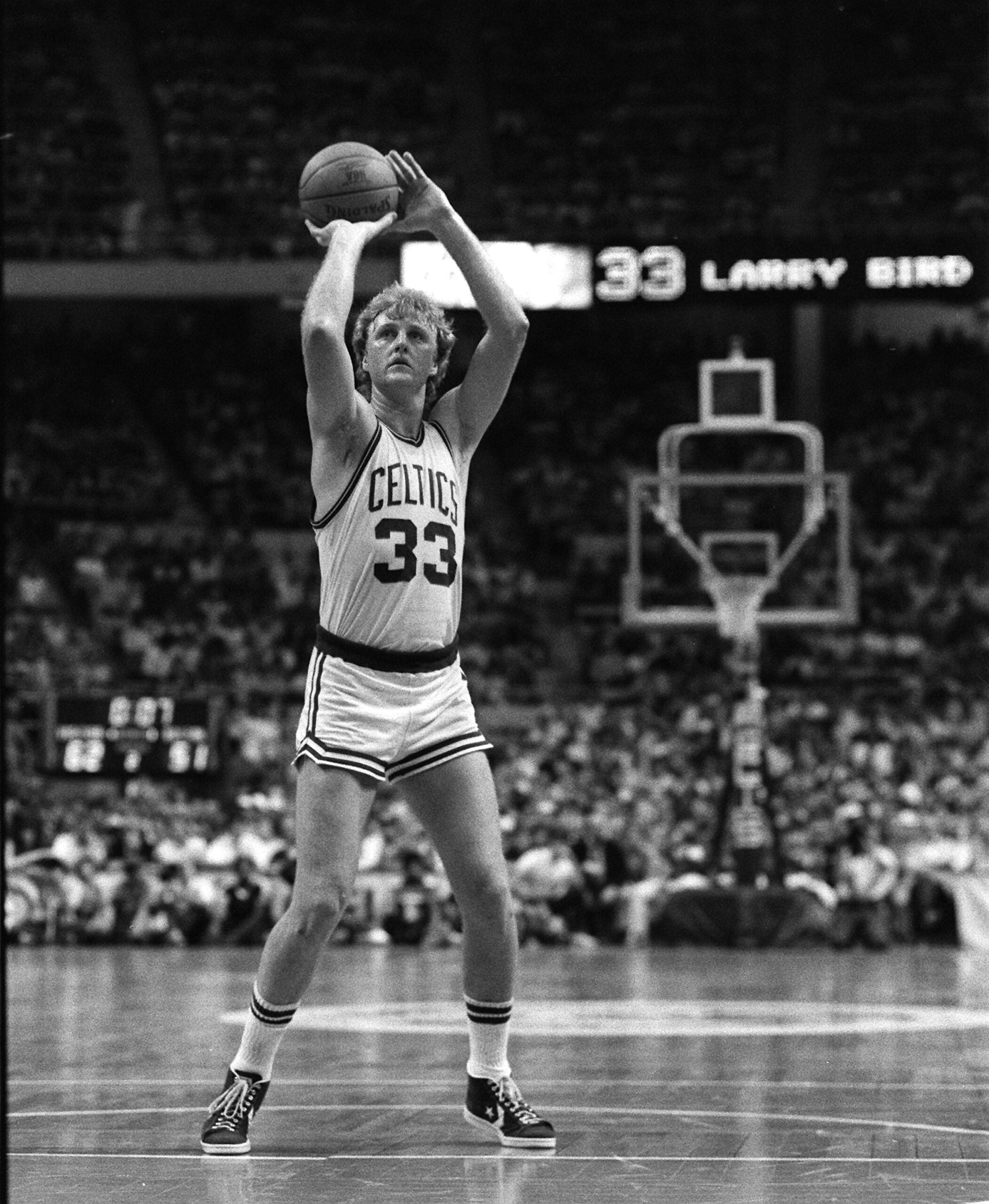This black-and-white photograph captures Larry Bird, number 33 of the Boston Celtics, poised to take a free throw on the basketball court, likely during a game or practice session at the Boston Garden. Clad in the iconic white Celtics uniform featuring green trim and his number 33, Bird stands on the free-throw line, ready to release the basketball held in his right hand while his left hand guides it. His tall, imposing frame and blonde hair make him stand out prominently. The background showcases a full house of spectators on the bleachers, although the crowd appears blurry and indistinct. The parquet floor and the distinctive Celtics symbol at midcourt, along with the scoreboard displaying Bird's number, further anchor the scene within the Boston Garden.